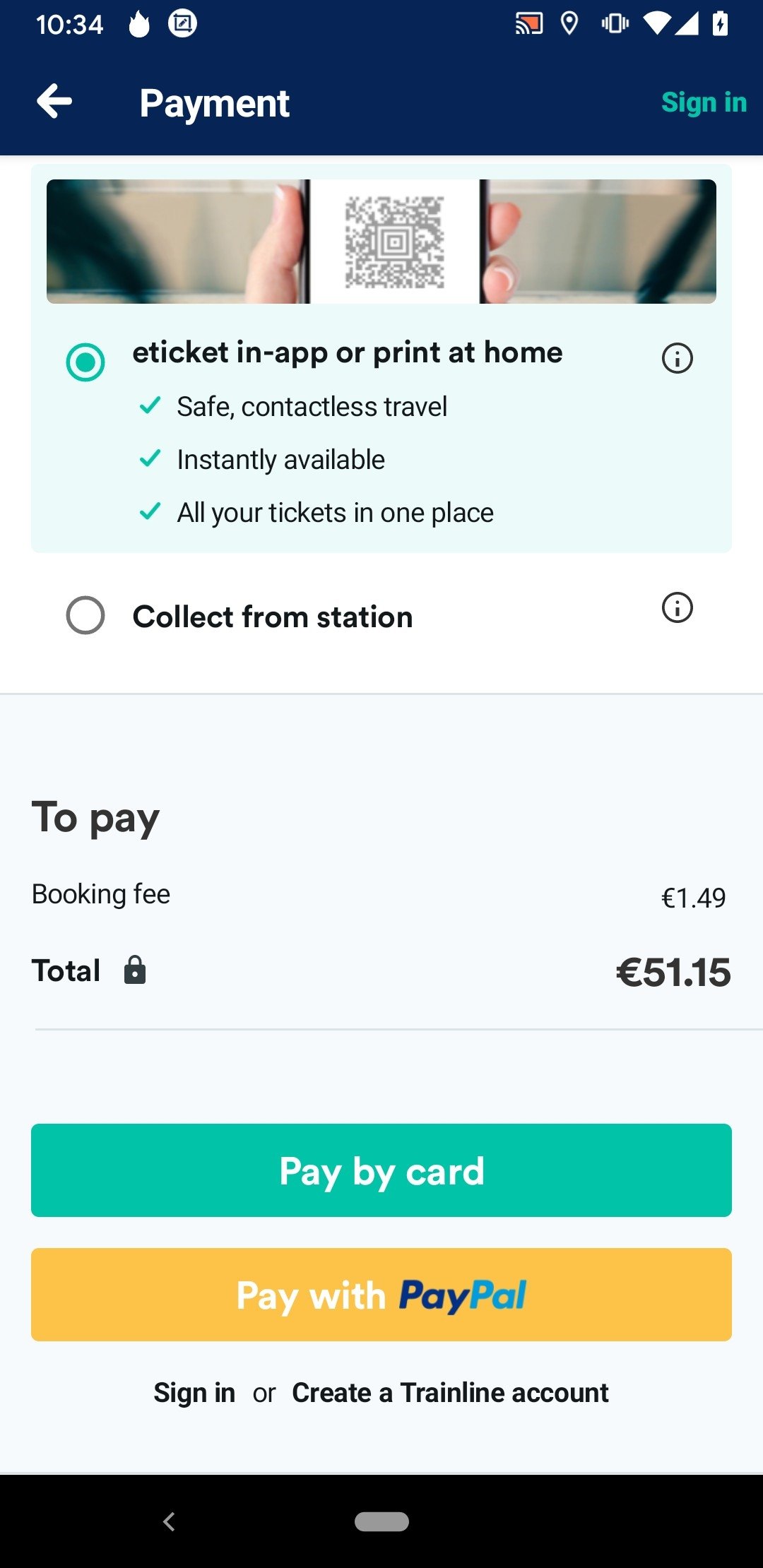This descriptive caption provides a thorough and detailed walkthrough of the various elements visible on a phone screen displaying a payment interface. 

---

**Detailed Caption:**
The image displays a phone screen in portrait mode, showcasing a payment interface. At the top, within a blue section, the time "10:34" is displayed on the left, alongside a small flame icon and a white circle containing a blue square. To the right, there are icons indicating screen recording status, Wi-Fi connectivity, and reception strength, as well as a marker icon. 

Directly below this section, there is a white arrow pointing left labeled "Payment" in white text, and a green "Sign In" text on the right. In the main portion of the screen, a QR code is being held up by a hand. Below the QR code, text reads "E-ticket in app or print at home," followed by three bullet points with checkmarks, listing features: "Safe contactless travel," "Instantly available," and "All your tickets in one place."

Among the options displayed, there's a green tick-marked button to "Collect from station" and details about a booking fee of 1.49 euros. The total amount due is listed as 51.15 euros, accompanied by a lock icon.

At the bottom of the screen, there are two payment options: a green "Pay by card" button and a yellow "Pay with PayPal" button. Additionally, text in black indicates the option to "Sign in or create a Trainline account." The screen ends with a black bar at the very bottom.

---